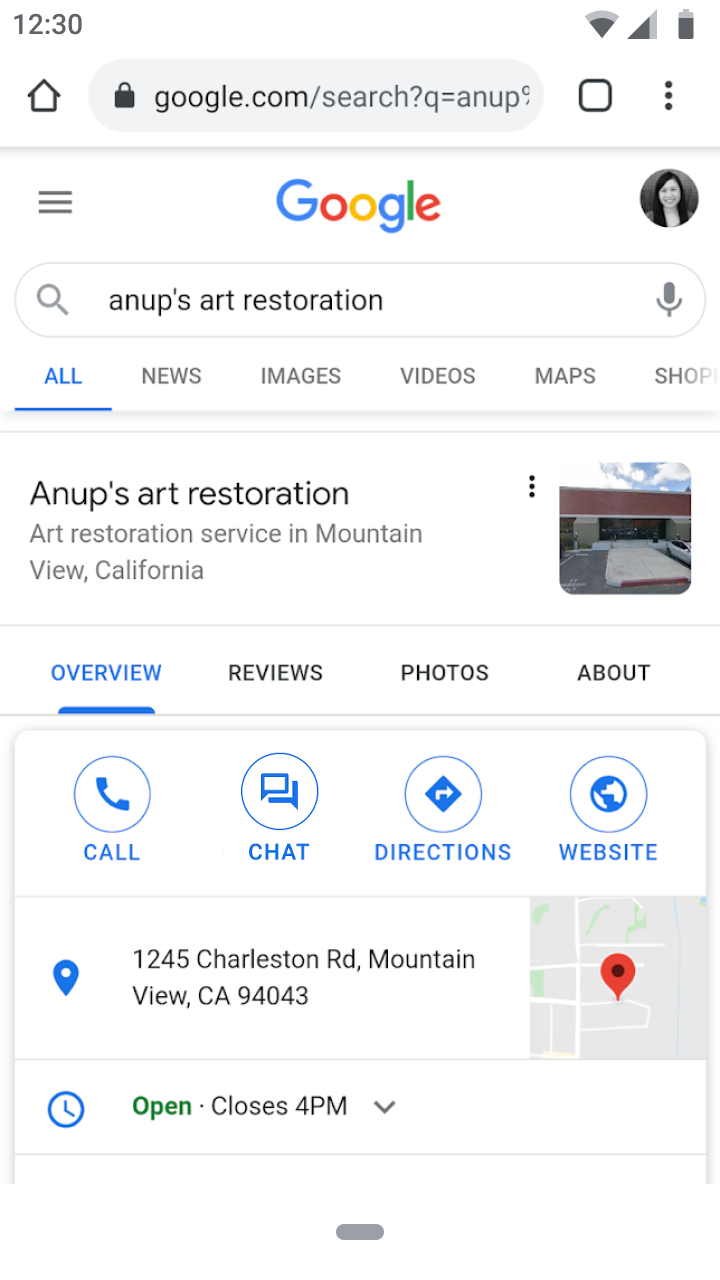Screenshot of a Google Search Result on a Smartphone

The screenshot captures the Google homepage on a smartphone, shown at 12:30 PM. The status bar at the top right corner displays the Wi-Fi and battery icons. Below the status bar are the home icon and search bar.

In the main content area, the Google logo is prominently displayed alongside a profile photo of a user. Underneath, there's a search box containing the query "Anup's art restoration" and a microphone icon on the right side.

Tabs for navigating different types of search results—All (currently selected), News, Images, Videos, Maps, and Shopping—are situated below the search box. Following these tabs is the top search result for "Anup's art restoration," labeled as an "Art Restoration Service in Mountain View, California," accompanied by a photo of the service's brick-and-mortar store and three vertical dots for additional options.

Further down, there are navigation tabs for Overview (selected), Reviews, Photos, and About related to the search result. Action icons for phone, chat, directions, and the website are also displayed. A map snippet with a location marker appears, pinpointing the address at 1245 Charleston Road, Mountain View, California, 94043.

The service's operational status is indicated with an 'open now' note, showing that it closes at 4 PM, with additional details accessible via a drop-down arrow. The bottom of the screenshot features the home button for quick exit.

---
I retained the important elements, labeled them clearly and in order, while avoiding repetitiveness. If you need more technical aspects included or a different angle, let me know!